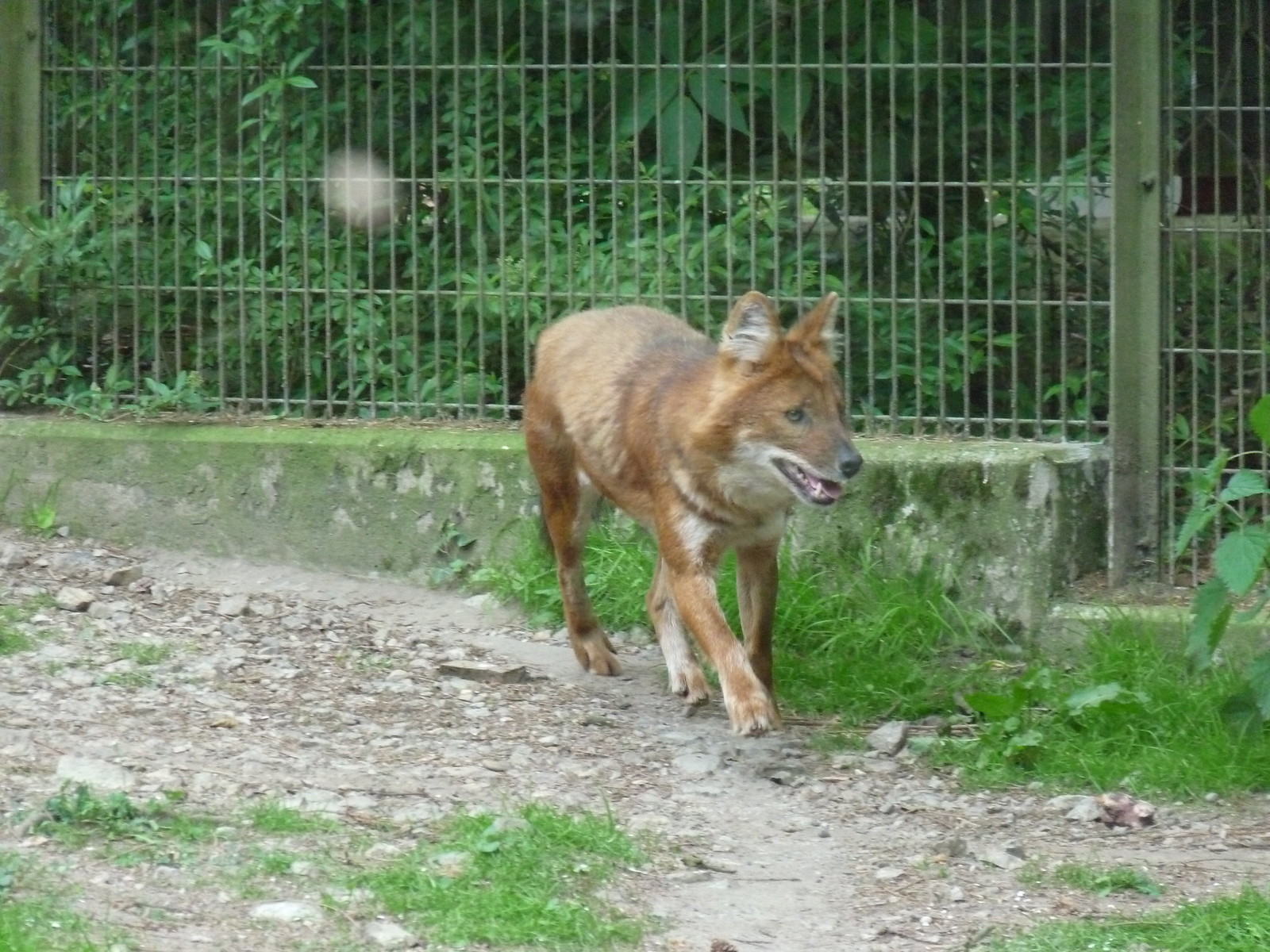The photograph features a small mammal, likely a fox or coyote, walking in an enclosure or cage. The animal has a rich, dark gold to orange coat with some white and darker, black spots. It has a black snout, a white muzzle extending to its chest, white markings in its pointed ears, and white patches on its legs. The animal's mouth is open, revealing its white teeth and pink tongue as it appears to be panting and looking off to the right. The enclosure's floor is a gravelly dirt path with dry soil, patches of vibrant green grass and plants scattered around. In the background, there is a green metal fence with posts, designed to keep wildlife out, and beyond the enclosure, there are more trees and vegetation with green moss growing on a cement wall.